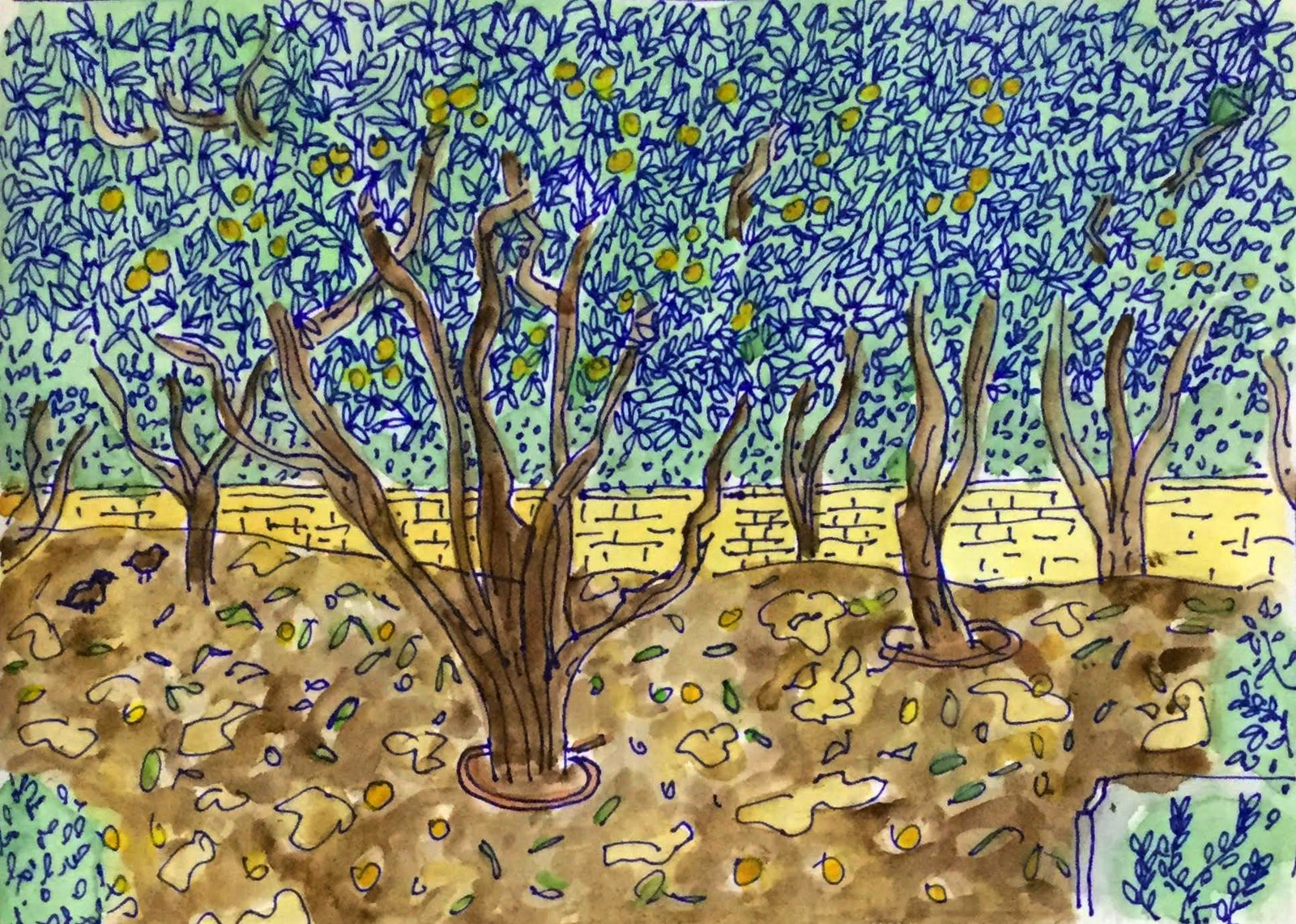This is a child's intricately detailed art project, possibly created with marker pens or watercolors. The artwork depicts a unique outdoor scene featuring a barren, brown field scattered with various forms of refuse such as spent fruit, leaves, and even items that resemble shirts. Prominently, the field contains several vine-like trees, each with brown trunks and dark outlines, adorned with numerous blue leaves and flowers. The tops of the trees are densely covered with these blue flowers, numbering at least a hundred or more, creating a vibrant canopy.

Interspersed within the foliage are clusters of yellow and orange circles, likely representing different fruits such as oranges, lemons, or apples. These fruits also appear scattered across the ground, adding to the mismatched array of objects on the field. In the lower right-hand and left-hand corners, green shrubs or bushes contribute additional texture to the scene.

The background features a short, tan, rock wall running horizontally across the middle of the image, providing a clear demarcation between the foreground and background. Two birds sit on the ground, enhancing the lively but slightly chaotic ambiance. The sky above the scene is a greenish-blue hue, complementing the earthy tones below while adding another layer of color to this imaginative landscape.